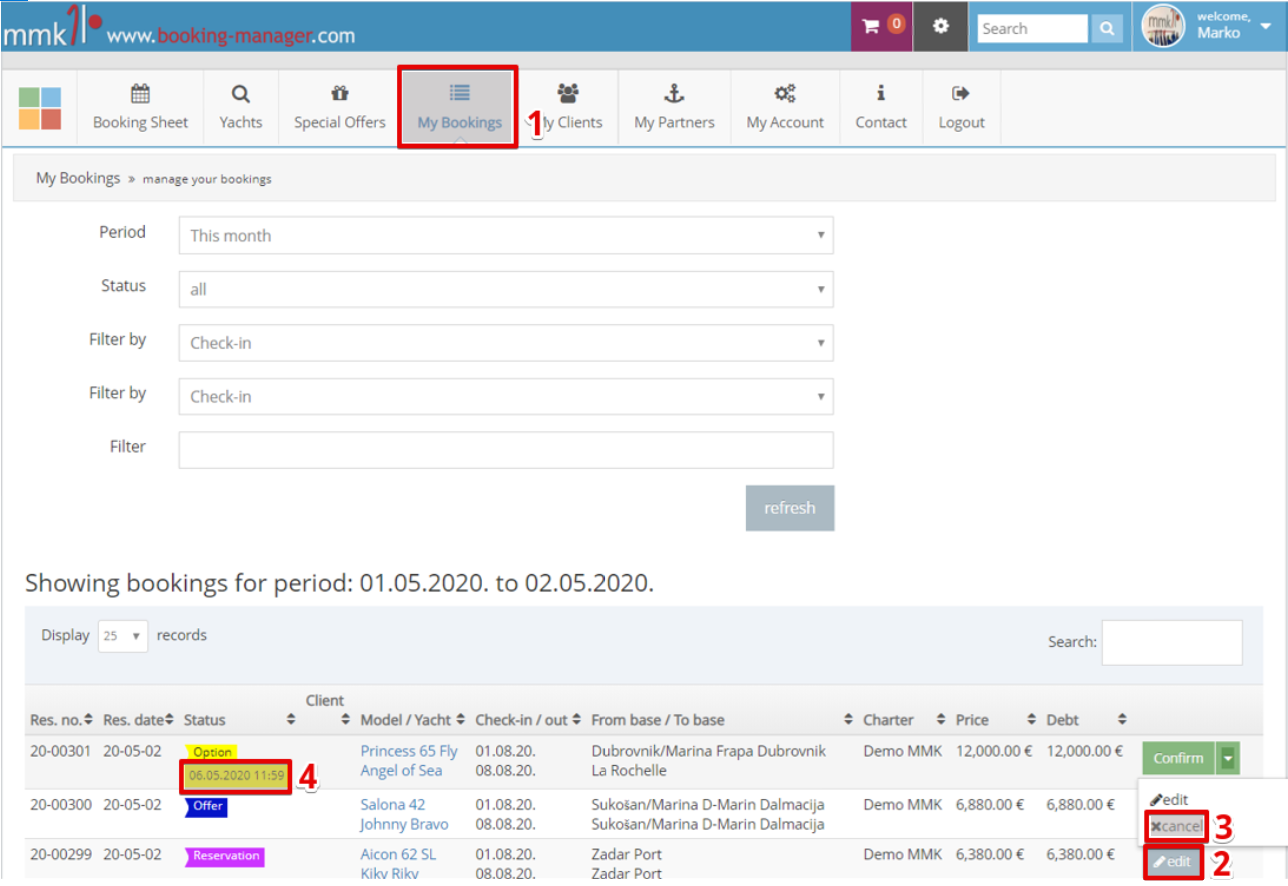This image is sourced from www.bookingmanager.com, depicting a user interface of a booking management application. The screen in focus is labeled "My Bookings - Manage Your Bookings." The interface includes multiple dialog boxes allowing users to input various parameters such as period, status, and filters to tailor their search. At the bottom, a section titled "Show Bookings for Period January 5, 2020 to February 5, 2020" lists three bookings. Each booking entry provides detailed information including check-in and check-out dates, price, and additional relevant details.